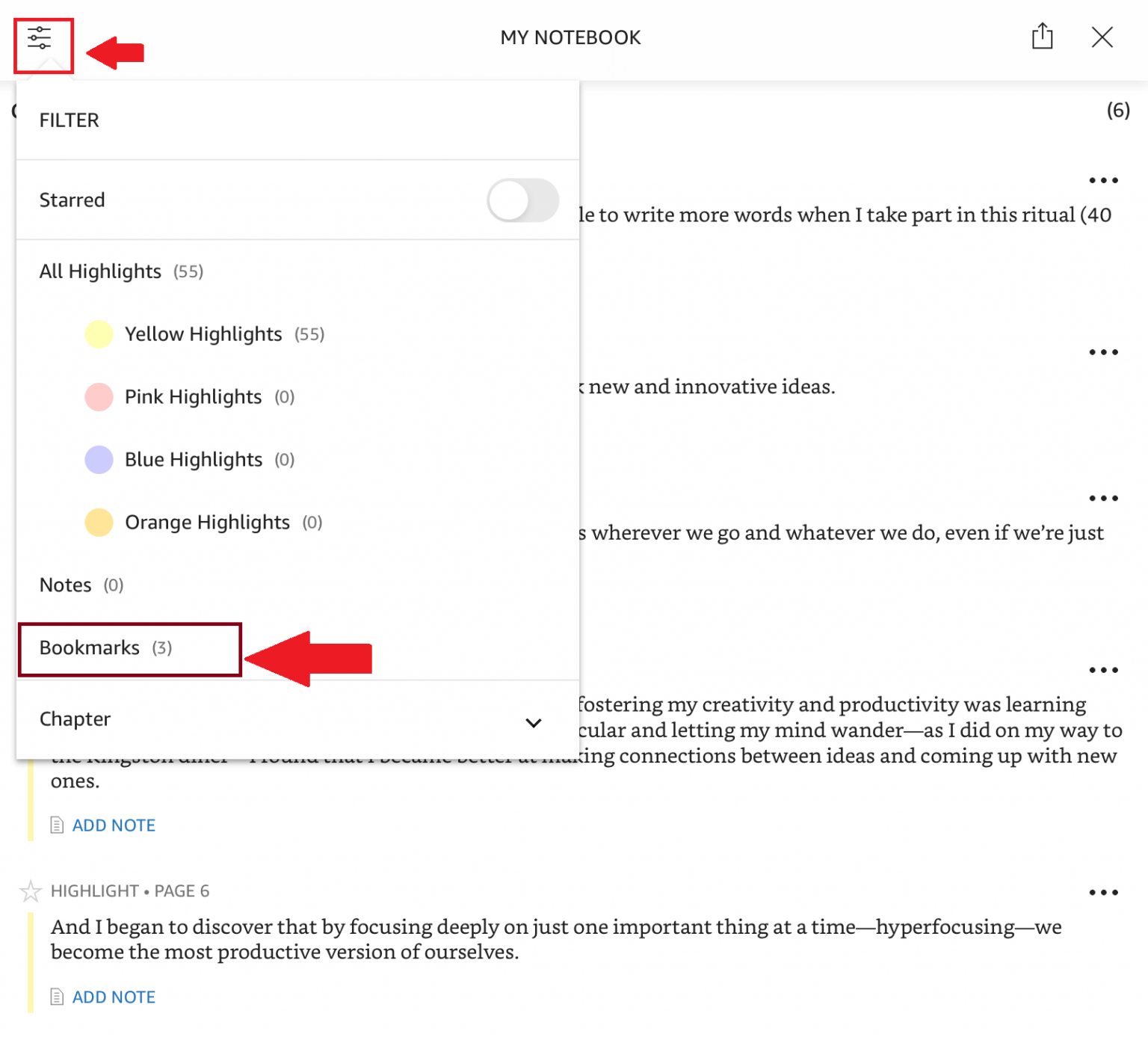On a plain white background, a digital notebook interface is prominently displayed. The title "My Notebook" is evident at the top center. On the left side, there is a navigation menu featuring three horizontal lines, each with dots scattered across them. These lines are surrounded by a red box and highlighted with a red arrow pointing towards them, suggesting an interactive element or important feature.

Just below the navigation menu, a section labeled "Bookmarks (3)" is marked with another red box and red arrow, drawing attention to it. The bookmarks section appears to be part of a dropdown menu that includes options such as "Filter Starred," with a toggle switch currently set to off, followed by different highlight color options: yellow, pink, blue, and orange. The menu also includes sections for "Notes," "Bookmarks," and "Chapter," the latter featuring a dropdown option.

The right section of the display features notes and content from the notebook, although the left-side menu partially obscures it, making it difficult to fully interpret. One visible note states: “Highlight Page 6: I began to discover that by focusing deeply on just one important thing at a time, hyper-focusing, we become the most productive version of ourselves.” Beneath this note, an “Add Note” button is present, suggesting functionality for adding further annotations.

Overall, the image depicts someone engaging with their digital notebook, utilizing various features such as highlights, bookmarks, and notes, possibly for the purpose of organizing and focusing their study or work efforts.